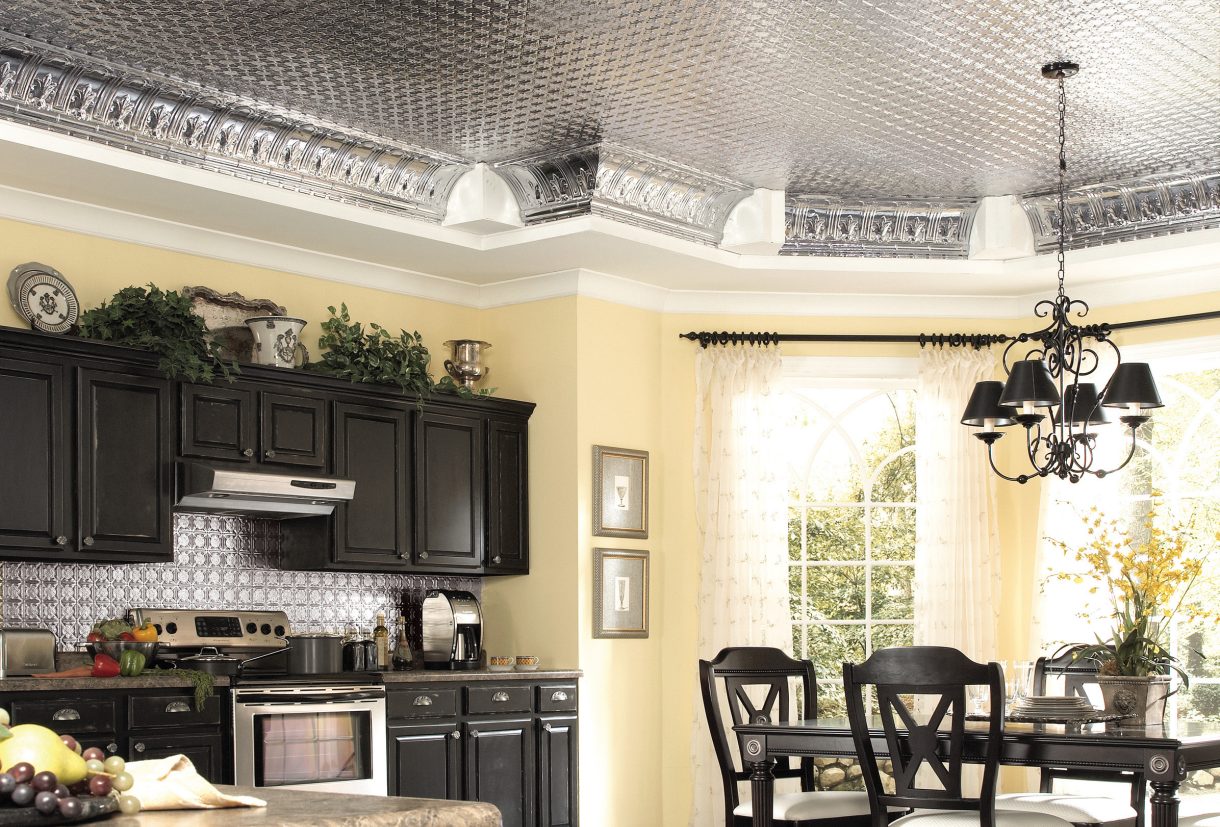This photograph captures a modern kitchen and dining area bathed in natural light. The kitchen features sleek, dark brown, chocolate-colored cabinets both above and below the countertop, topped with a stylish silver backsplash. An elegant stainless steel oven occupies a central spot in the kitchen, accompanied by various pots and decorative items, including a row of plants atop the cabinets. The light lemon, almost beige, walls of the room add a bright yet warm ambiance, complemented by the two open windows adorned with delicate white curtains. 

A striking feature of the room is its ceiling, covered in a beautiful, iridescent, silver metallic material with intricate moldings, adding a touch of sophistication. Hanging from this ceiling is an ornate black pendant light, which gracefully illuminates the sturdy dining table below. This table, glass-topped with a brown frame, is accompanied by four black, chocolate-colored chairs, each with a white cushion, offering a comfortable and stylish seating arrangement. To the left of the dining area and near the kitchen island, which also sports grapes and other fruits, are two framed photos adding a touch of personal flair to the chic and well-organized space.